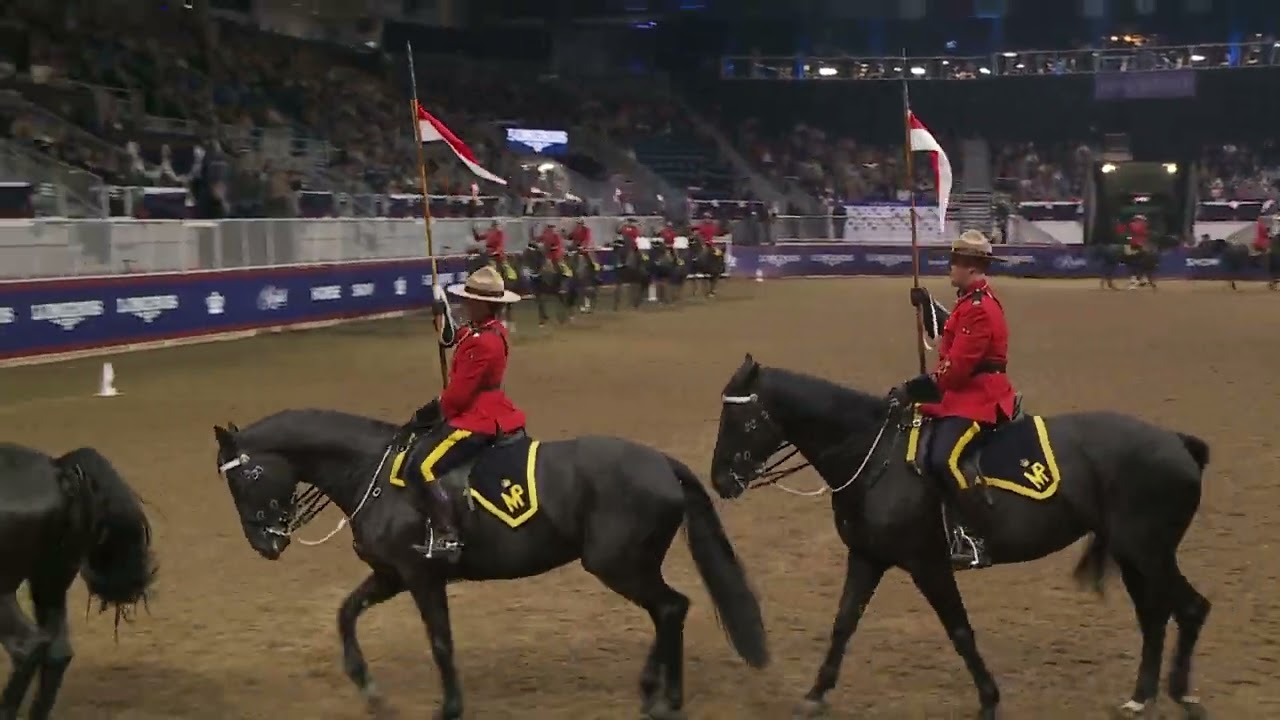In this detailed photograph taken within a large stadium or arena, the focus is on a group of Canadian mounted military police officers parading on well-groomed, black horses. The arena's floor is a dirt surface, with a purple banner encircling its perimeter and a white metal fence above that, leading up to the stands teeming with slightly blurred spectators. In the foreground, two officers, moving towards the left, are prominently visible on their horses. They are dressed in striking, traditional uniforms: bright red jackets, black pants with a yellow stripe along the sides, black gloves, and tan hats with black bands. Each officer holds an American flag mounted on a wooden pole in their right hand, and some also carry red and white flags. The horses are adorned with black blankets bordered in gold, emblazoned with the letters "MP" in gold. The horses also feature black and white bridles and bits. Additional officers, dressed similarly, are visible further back, forming an organized row and some facing the right. The stadium wall is adorned with blue banners that appear to have white lettering, possibly spelling out "Longhorns," though the text is slightly blurred. This captivating scene exudes regality and precision, catching the disciplined elegance of the mounted officers and their majestic horses.